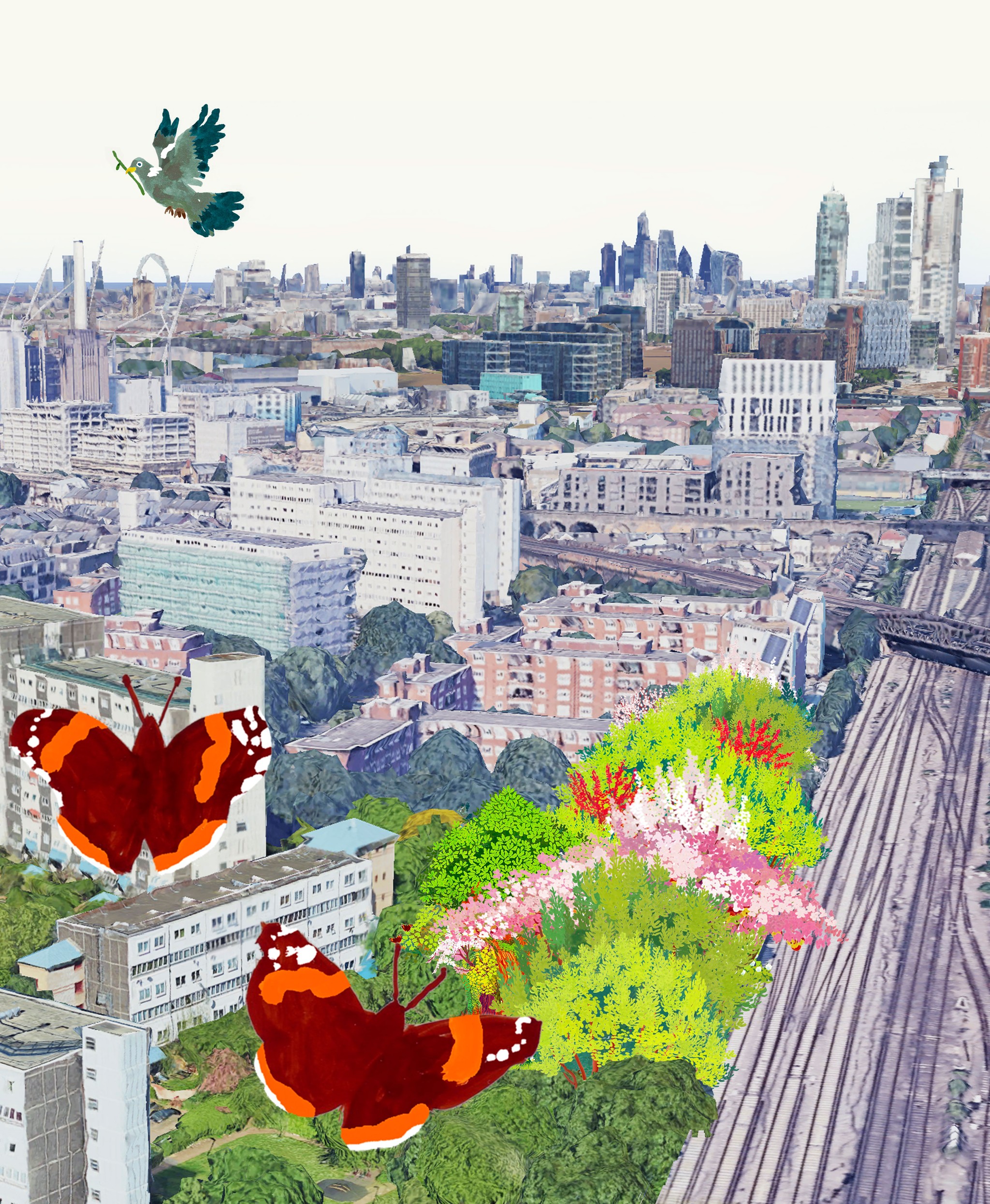The painting, titled "Heritage Forest," offers a detailed aerial view of a city skyline, blending natural elements with urban structures. Dominating the right side is a pink highway with white and purple lines, ascending diagonally. The lower segment features dense vegetation, including dark and light green bushes, a pink and purple-leaved plant, and a bush adorned with striking red leaves. Central to the image is a cream-colored, hospital-like building with a flat roof, surrounded by several towering structures—one notably white, and another with a teal facade. The distant background reveals more tall buildings, particularly a light teal one with square windows on the right.

Noteworthy is a large, vibrant green bird with dark green wingtips, a white eye, and a yellow beak, soaring in the upper left corner, symbolically holding a branch. Nearby, two oversized butterflies with orange bodies, light orange wing stripes, white wing dots, and orange-tipped antennas float above the bottom left, adding a dramatic splash of color. The painting creatively juxtaposes the city's gray and blue hues with these vivid natural elements, emphasizing the harmonious, yet contrasting coexistence of urban and natural environments.